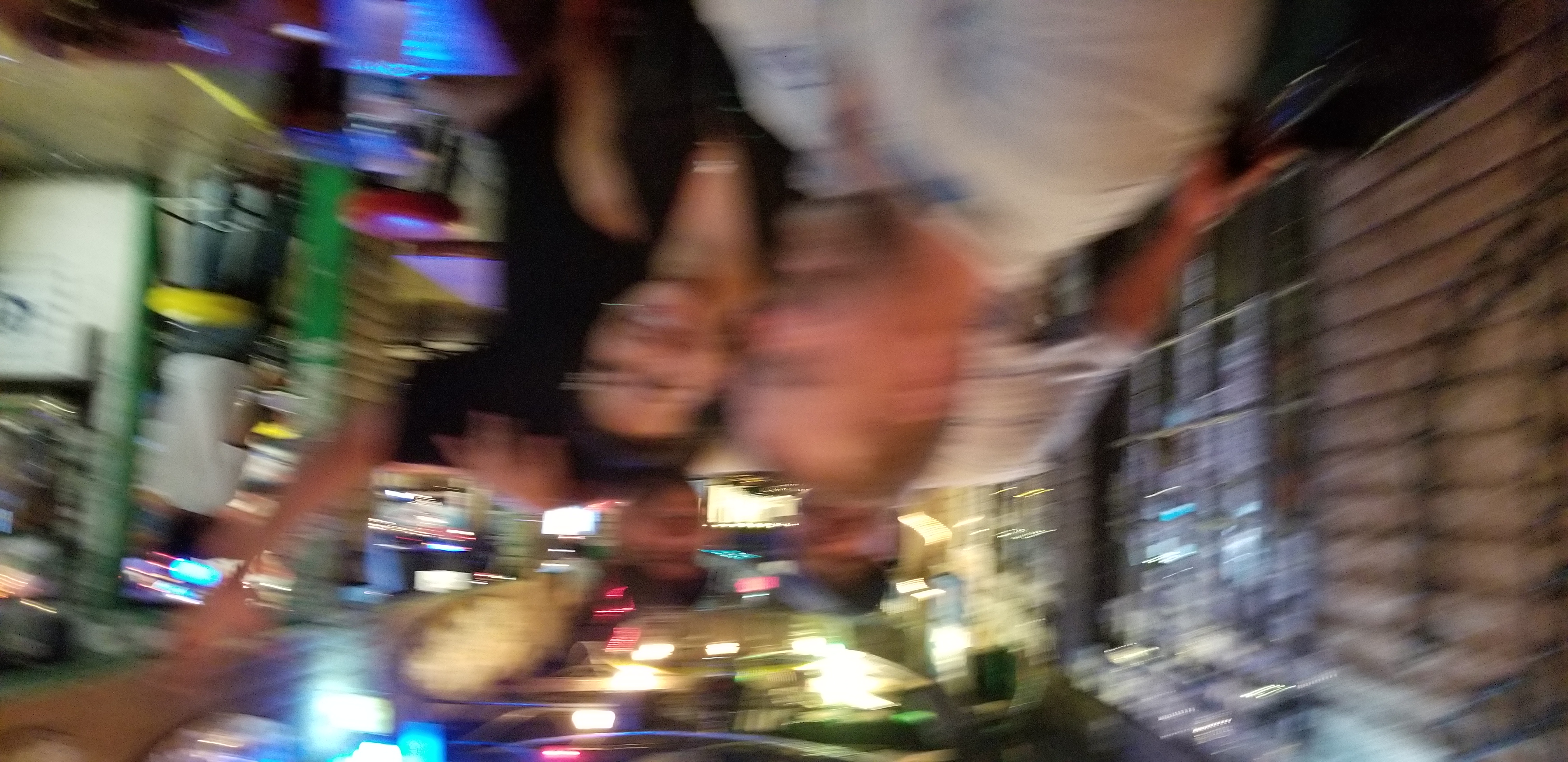A highly blurred and upside-down photograph appears to capture four individuals in an urban nighttime setting. Two men, possibly wearing hats, stand towards the back, while in the foreground, a man with very short, reddish-brown hair, dressed in a white shirt, sits next to a woman. The woman, who has dark hair and wears glasses, is clad in black attire. The backdrop reveals a cityscape with illuminated buildings, suggesting they might be near a gas station or similar establishment.